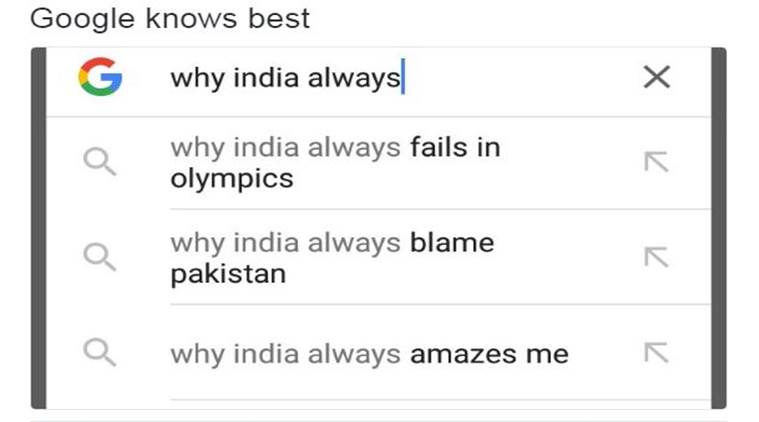This meme is a cropped screenshot of Google search results, focusing on the quirky and often humorous autocomplete suggestions. At the top left, the Google logo—a stylized "G"—is prominently visible next to the search bar, which contains the partially typed phrase "why India always." Below this, the autocomplete feature displays a list of popular search queries, including:

1. "why India always fails in Olympics"
2. "why India always blame Pakistan"
3. "why India always amazes me"

Each search suggestion is accompanied by a magnifying glass icon on the left, indicating that clicking it will perform that specific search. To the right of each search entry, there is an upward-pointing diagonal arrow, providing options to erase that particular suggestion. The top right corner of the search bar also features a small "X" for clearing the search input.

At the very top of the meme, the text "Google always knows best" is prominently displayed, humorously highlighting Google's predictive capabilities. The overall background of this image includes vertical gray boxes on both the left and right sides, revealing that the meme was cropped from a larger screenshot with a gray backdrop.